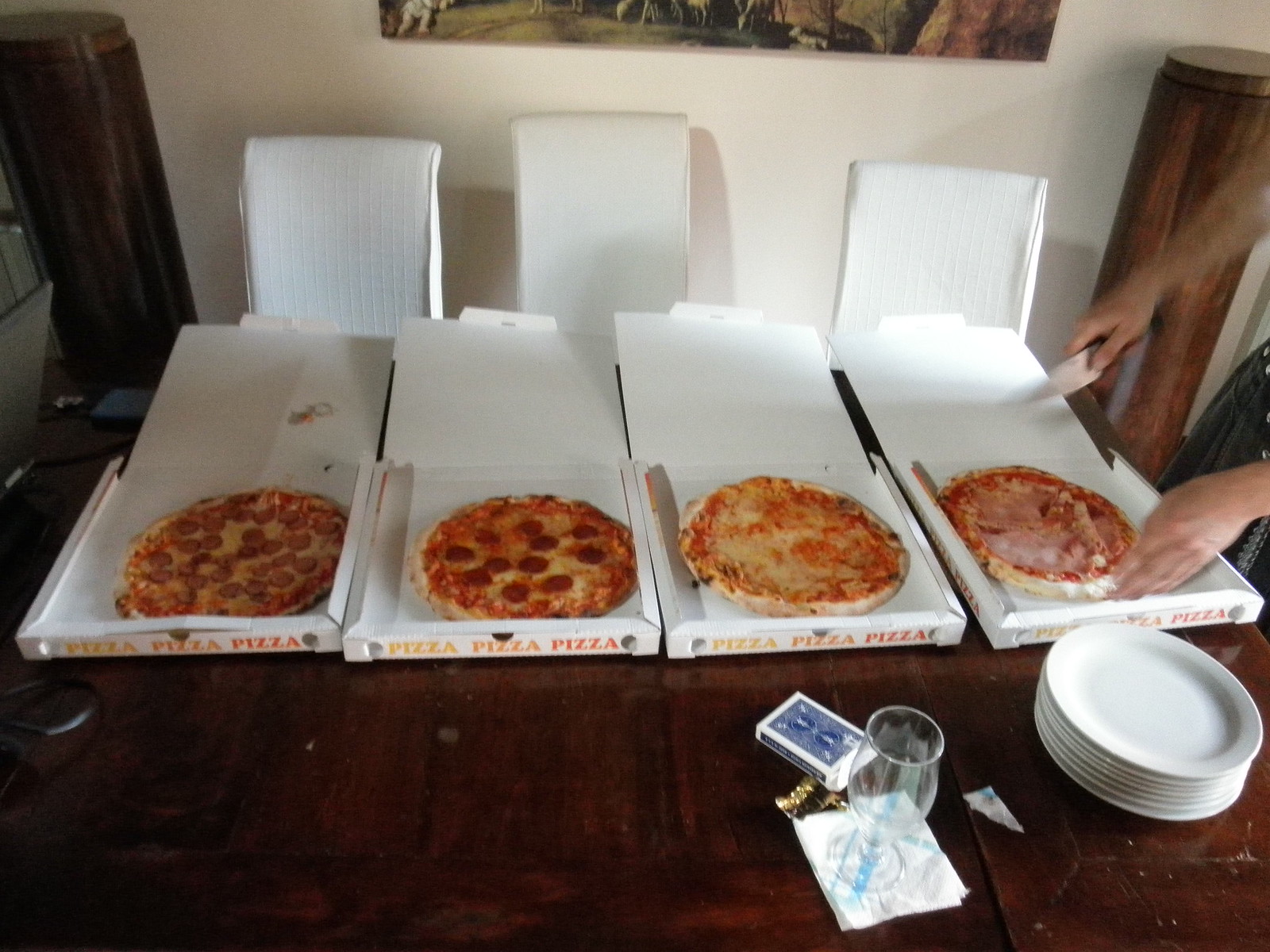In this photo, we see a cozy pizza lunch set up inside someone's home on a polished, dark wooden table. The table features four open white pizza boxes, each emblazoned with "pizza" in colorful letters (yellow, orange, and red) along the bottom edge facing the camera. To the left, two boxes display mouth-watering pepperoni pizzas, while the two on the right contain primarily cheese pizzas. Behind these boxes, there appear to be additional pizzas partially obscured by the open lids. In the foreground, a neat stack of small white paper plates is ready for serving, accompanied by a clear wine glass placed on a white cocktail napkin with a blue design. A small deck of playing cards and some indistinguishable items, possibly keys, also rest on the napkin. In the upper right corner, a blurred, motion-captured set of hands—likely a woman’s—cuts into one of the cheese pizzas, adding a dynamic touch to the scene. The atmosphere suggests a laid-back, intimate gathering surrounded by simple, yet thoughtful details.